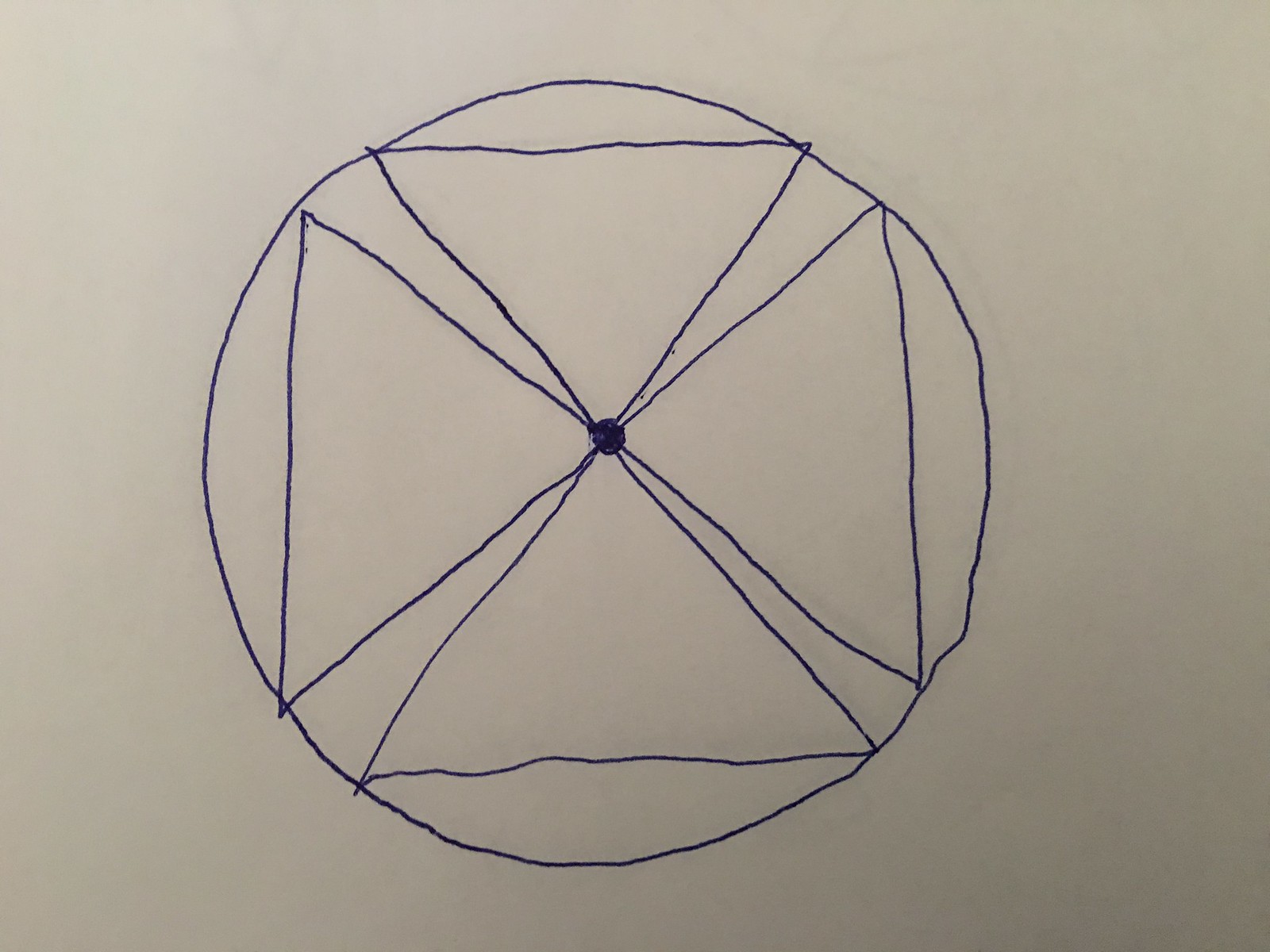In the image, there is a detailed sketch featuring a prominent circular shape outlined by a blue line. This circular boundary encloses a geometric arrangement comprising four narrow, dark blue lines forming an X pattern. These intersecting lines create a central grid-like design that can be interpreted either as four individual triangles or as a composite square. At the very center of this X pattern is a distinct, solid blue dot. The entire sketch is drawn on a light gray background, emphasizing the sharp contrast between the blue lines and the paper. The overall composition blends simplicity with intricate geometric design, capturing both linear and circular symmetry.